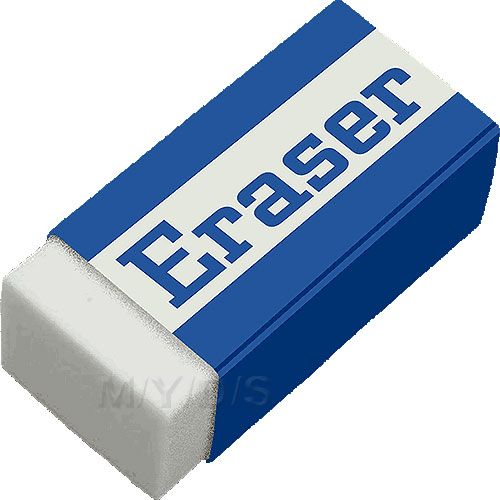The image features a photorealistic depiction of an eraser set against a completely white background. The eraser is placed diagonally, angling from the lower left to the upper right. The visible portion of the eraser shows a spongy white area on the left end, suggesting it might be intended for use on whiteboards rather than chalkboards. Covering the eraser is a blue plastic body with a white strip in the center. On this white section, the word "eraser" is printed in blue, with a capital 'E' followed by lowercase 'r', 'a', 's', 'e', 'r'. The image appears pixelated and includes a watermark reading "M/Y/D/S."